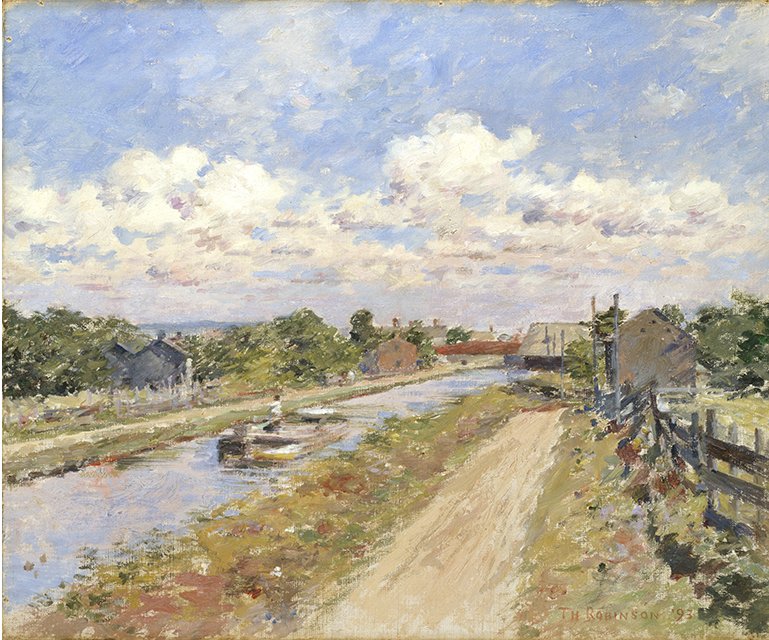The painting depicts a picturesque village scene on a bright and sunny day. The composition features a small canal running through the village, with a man navigating a boat down the waterway. To the left of the canal, there are several houses surrounded by lush trees and bushes, while a dirt path and a long wooden fence line the right side, where more houses can be seen further in the distance. The sky, which occupies almost half of the painting, is a vibrant blue filled with big, fluffy white clouds tinged with shades of gray and purple, reminiscent of a Monet-style impressionist work. The color palette includes black, white, gray, brown, yellow, green, blue, and a touch of purple. A signature in the bottom right corner reads "T.M. Robinson, 93," suggesting the artist and possible year of creation. The overall scene exudes tranquility, capturing the serene beauty of the village with impressionist strokes that prioritize color and atmosphere over fine detail.